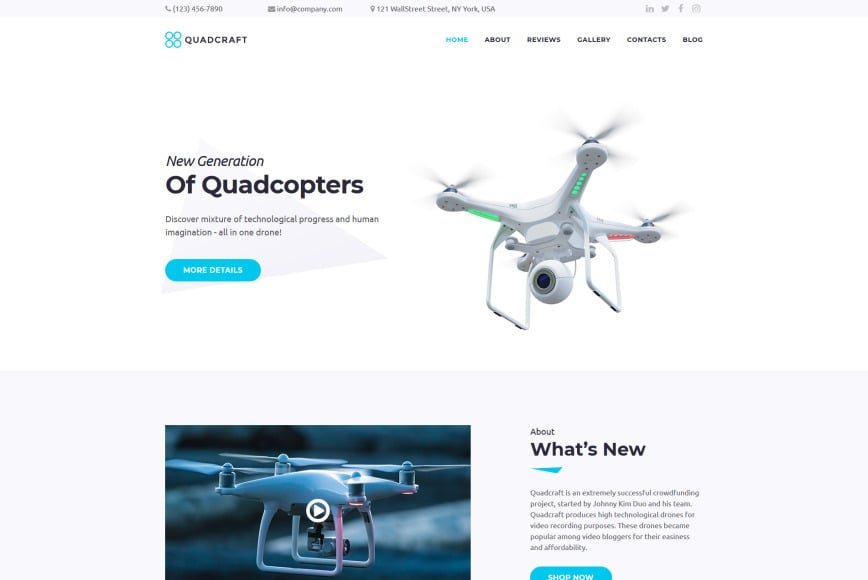This is a screen capture of the home page of a website named QuadCraft. The website name is prominently displayed in black text on the top left, accompanied by the company logo, which features four blue circles arranged in a square formation. 

The header menu of the website includes options such as Home, About, Reviews, Gallery, Contacts, and Blog. The Home section is currently selected, indicated by light blue text, while the other menu items are in black text.

On the right side of the page, there's an image showcasing the new generation of quadcopters. Accompanying the image, bold text reads "New Generation of Quadcopters," followed by a caption that states, "Discover a mixture of technological progress and human imagination all in one drone." Below this, there's a prominent button in bright blue with white text that reads "More Details."

Further down, the page features another section dedicated to this innovative quadcopter. On the left side, there is a video presentation about the quadcopter. Adjacent to the video on the right, bold black text introduces the section with the phrase "What's New." Beneath this heading is a detailed description of the quadcopter, written in grayish text, providing comprehensive information about the product's new features and capabilities.